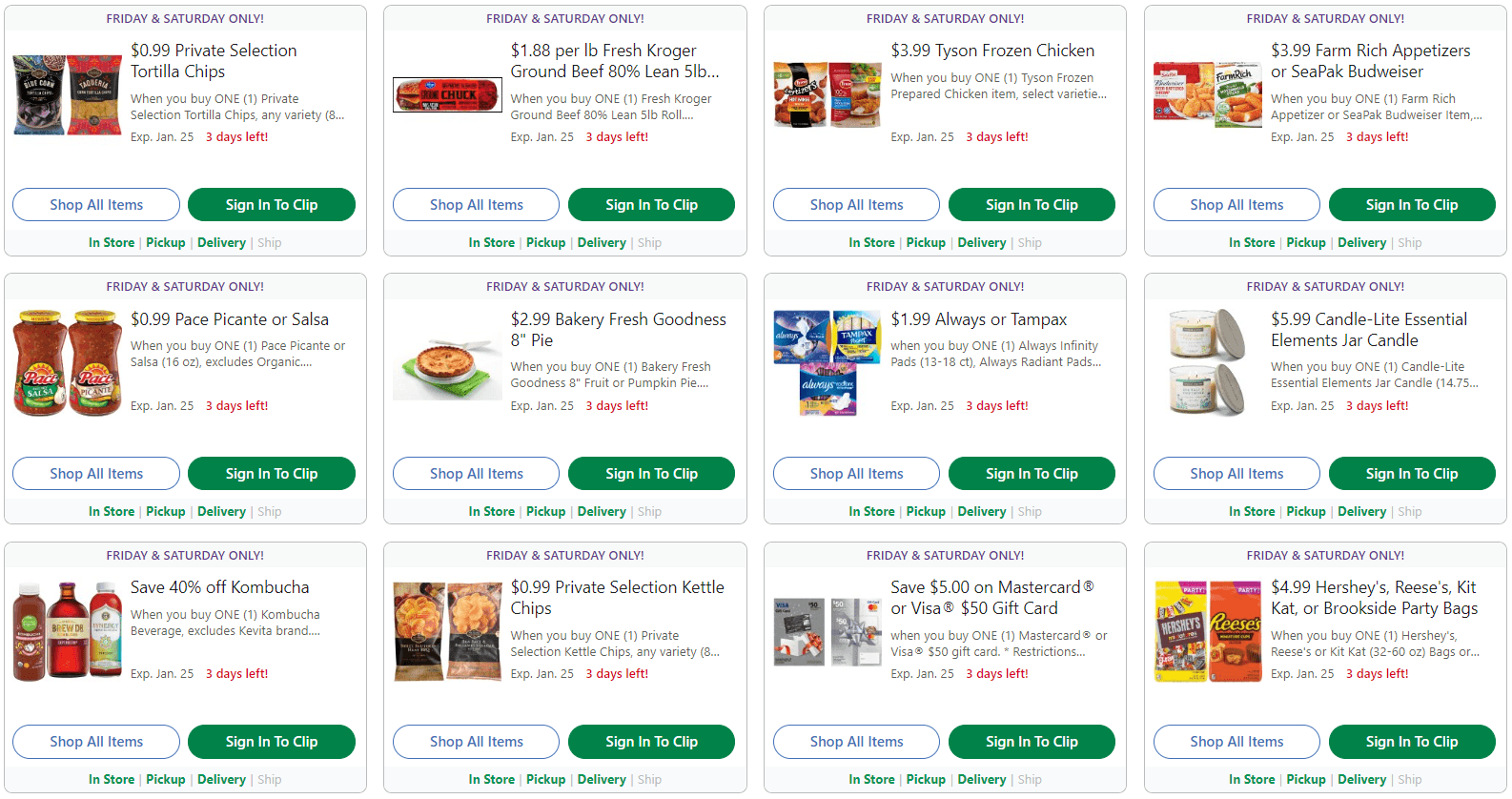The image is a screenshot from an opera website showcasing a selection of digital coupons organized into four columns, each containing three coupons. Each coupon is rectangular, predominantly white with gray bars at the top and bottom. 

At the top of each coupon, within the gray bar, the text "Friday and Saturday only" is displayed. Below the headline, each coupon includes two buttons: a white one with a blue border and blue text reading "Shop All Items," and a green one with white text reading "Sign In to Clip." At the bottom gray bar of each coupon are four options—In-Store, Pickup, Delivery, and Ship—with the Ship button grayed out.

### Column 1:
1. **99¢ Private Selection Tortilla Chips**
   - Offer: 99¢ for Private Selection Tortilla Chips, any variety, when you buy one.
2. **99¢ Pace Picante or Salsa**
   - Offer: 99¢ for 16-ounce Pace Picante or Salsa, when you buy one.
3. **40% off Kombucha**
   - Offer: 40% off on Kombucha.

### Column 2:
1. **$1.88 per pound Fresh Kroger Ground Beef**
   - Offer: $1.88 per pound for Fresh Kroger Ground Beef, 80% lean, in a 5-pound pack.
2. **$2.99 Bakery Fresh Goodness 8-inch Pie**
   - Offer: Bakery Fresh Goodness 8-inch Pie for $2.99.
3. **99¢ Private Selection Kettle Chips**
   - Offer: 99¢ for Private Selection Kettle Chips.

### Column 3:
1. **$3.99 Tyson Frozen Chicken**
   - Offer: Tyson Frozen Chicken for $3.99.
2. **$1.99 Always or Tampax**
   - Offer: Always or Tampax products for $1.99.
3. **Save $5 on MasterCard or Visa $50 Gift Card**
   - Offer: Save $5 when purchasing a MasterCard or Visa $50 gift card.

### Column 4:
1. **$3.99 Farm Rich Appetizers or CPAC Budweiser**
   - Offer: Farm Rich Appetizers or CPAC Budweiser for $3.99.
2. **$5.99 Candle Lite Essential Elements Jar Candle**
   - Offer: Candle Lite Essential Elements Jar Candle for $5.99.
3. **$4.99 Hershey's, Reese's, KitKat, or Brookside Party Bags**
   - Offer: Party bags of Hershey's, Reese's, KitKat, or Brookside for $4.99.